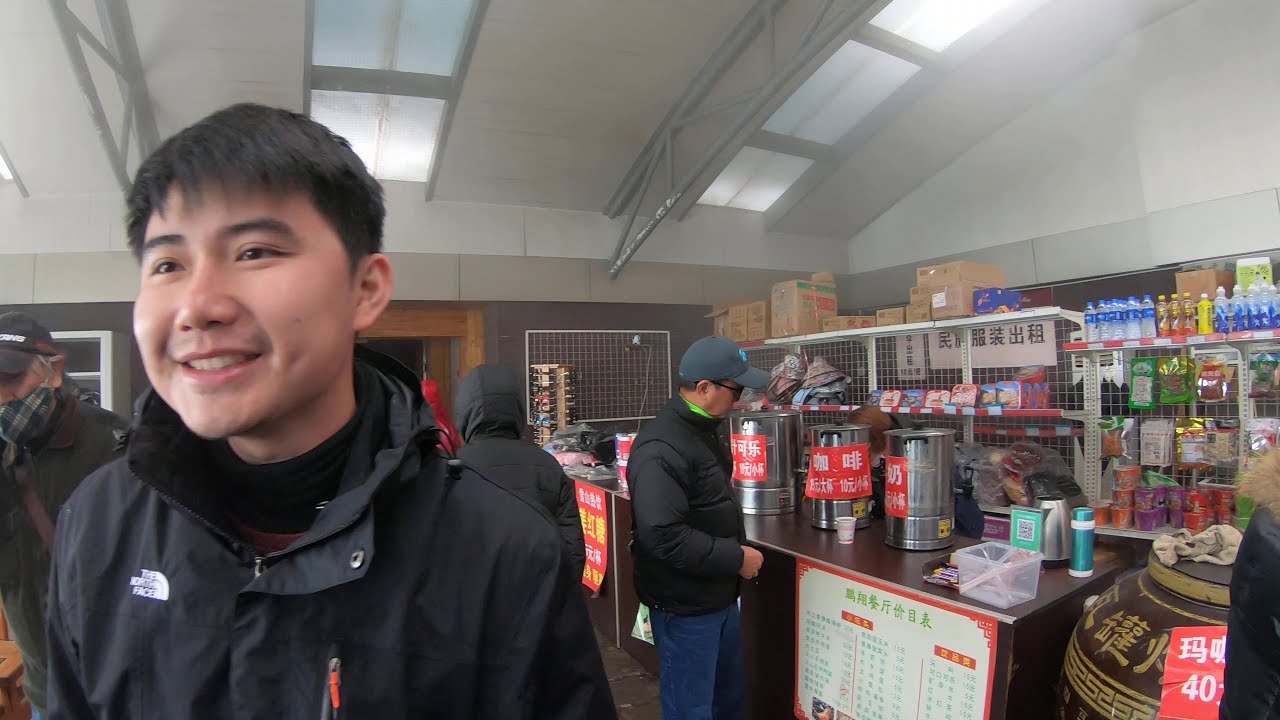In this detailed color photograph, taken in landscape orientation, the setting is a small, low-budget convenience store or coffee shop in an Asian country, identifiable by the abundance of signs and labels featuring Asian characters. The interior is modest with a white ceiling, black walls, and overhead rows of fluorescent lighting. 

On the left side of the image, a young Asian man, about 17 years old, stands smiling. He has short black hair and is dressed in a black zip-up jacket over a black shirt, with the collar of a maroon shirt just visible underneath. Behind him and slightly to his left is another man, also Asian, wearing a mask. 

In the foreground, there's a brown countertop displaying multiple tan cans with red labels featuring Asian characters, possibly in Chinese or Japanese. These items on the counter may include big silver pots containing some kind of liquid, perhaps soup, and there are condiments arranged to the right. A white sign with orange trim and Asian writing hangs off the table. On the shelves behind the counter, various packaged food items are neatly arranged, further lending to the impression of a convenience store setup. Additional signage with red backgrounds and white Asian characters is visible in the bottom right corner of the image. The photograph is a realistic representation of everyday life in this small store.